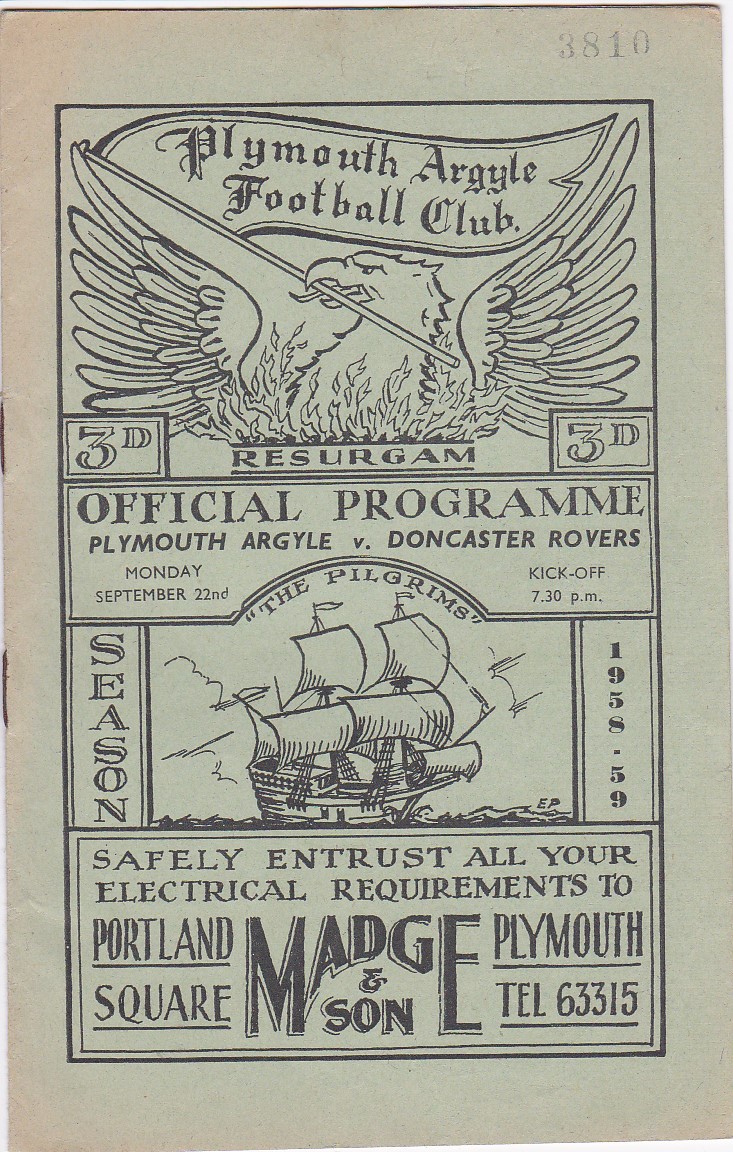The image appears to be an official program cover for a historic soccer match between Plymouth Argyle Football Club and Doncaster Rovers, scheduled for Monday, September 22nd, with a kickoff at 7:30 p.m. for the 1958-1959 season. Dominating the top of the image, the text "Plymouth Argyle Football Club" is prominently displayed alongside an emblem featuring an eagle with spread wings, holding a flag that reads "Plymouth Argyle Football Club." Below this, the details of the match are clearly stated, and next to them, there is a sketch of the Mayflower ship, complete with a cluster of flags billowing from its masts. The ship is captioned "The Pilgrims" in quotation marks, referencing the club's nickname. Adding to the nostalgic feel, an advertisement at the bottom advises readers to "safely entrust all your electrical requirements to Portland Square Madge and Son," providing their Plymouth telephone number, 63315. The entire imagery and text appear on an aged, beige-colored paper, enhancing the vintage appeal of the program.